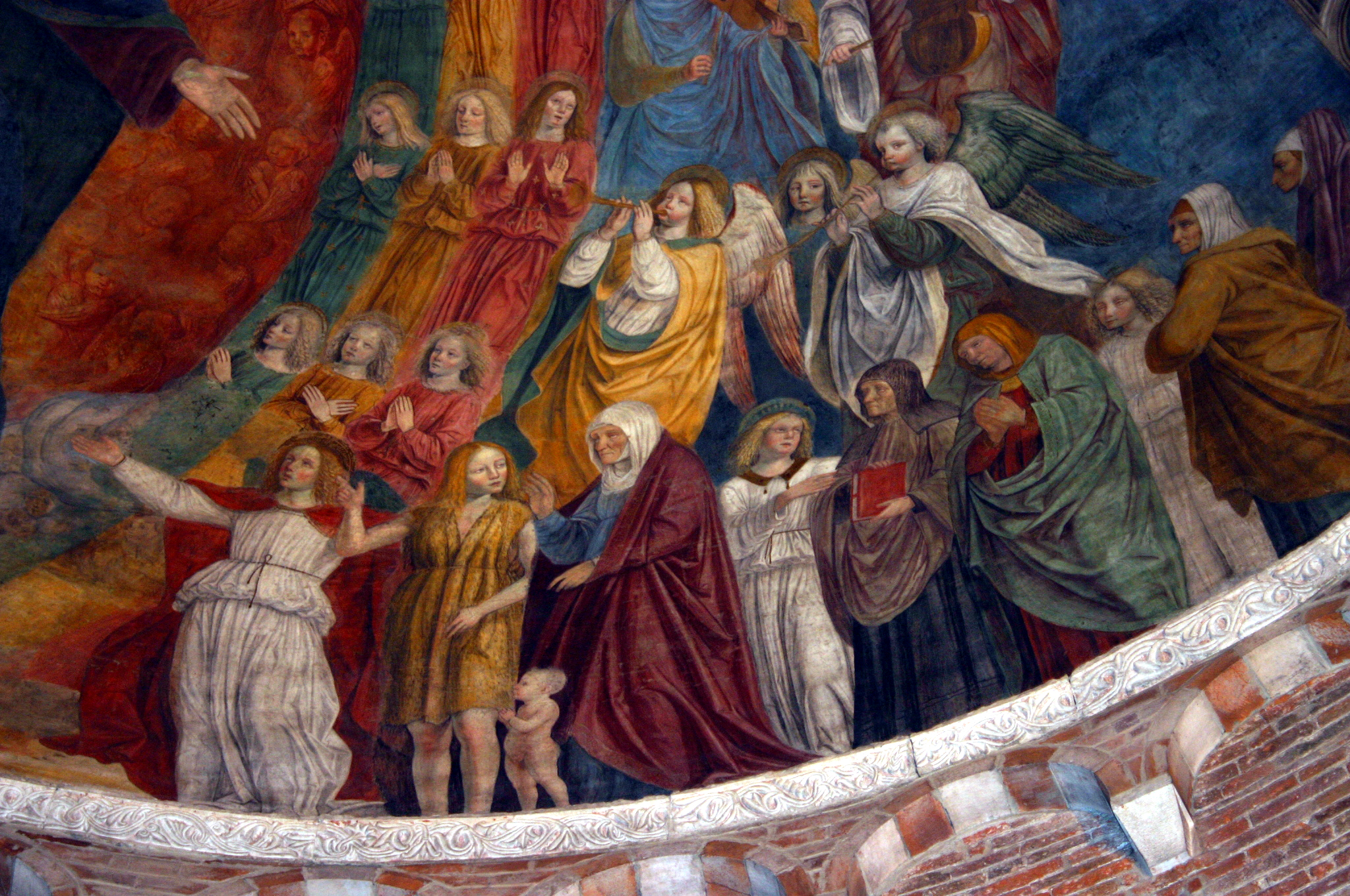The image is a detailed oil painting, likely a mural on the ceiling of a church, depicting a vibrant and historical scene. The foreground prominently features a red brick wall with a white cement top that slopes from the middle right to the bottom left, where a procession of about eight people is standing. These figures are adorned in varied, colorful robes and headdresses in hues such as crimson, light gray, yellow, green, purple, and brown. Among them, a naked baby is seen clutching its mother's dress. In the background, a religious ambiance is evoked with a blend of blue and other various colors painted on the walls. Above this scene, a choir and three angels, including one playing a flute, are depicted. To the left, three women in different colored dresses—red, rust, and green—are praying, with one holding her hands out and another looking down with her hands crossed over her chest. Below these figures, more women are kneeling in prayer, enhancing the painting's serene, devotional atmosphere.